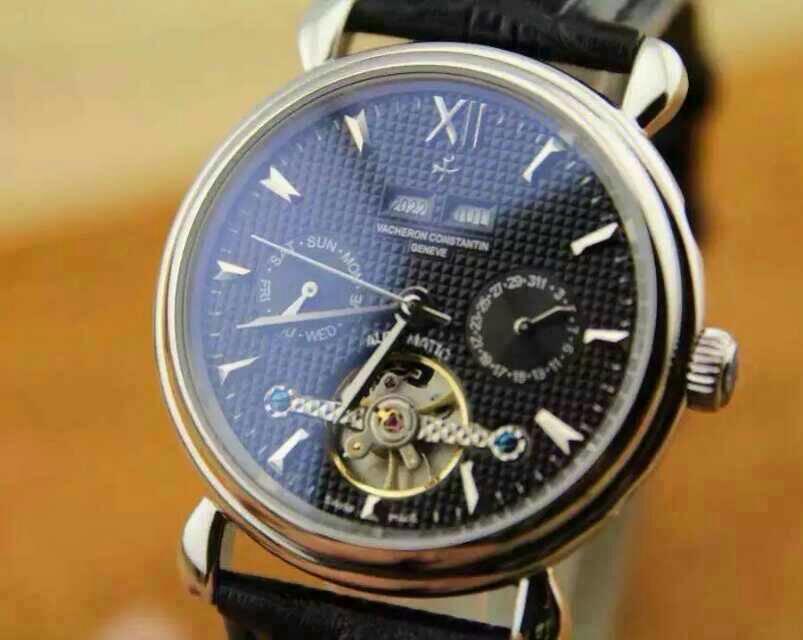This is a square color photograph showcasing a luxurious Swiss wristwatch by Vacheron Constantin. Positioned vertically in the center, the watch is set against a dynamic background that transitions diagonally from a lighter beige and yellow-orange in the upper left to a darker rust-orange in the lower right. The watch features a polished gold casing and a face adorned with intricate mini black squares. At the 12 o'clock position, marked with a gold Roman numeral, an emblem resembling a cross with cuneiform-like triangular points lies just below. The rest of the time indicators are represented by raised gold hash marks. This timepiece boasts three auxiliary dials forming an upside-down triangle: the circle at 9 o'clock shows the day of the week, the circle at 6 o'clock reveals the inner mechanics, and the function of the circle at 3 o'clock remains unclear. Additionally, the date is prominently displayed beneath the watchmaker's name, inscribed as "Vacheron Constantin Genève." The timepieces' black leather strap subtly extends into the frame, further emphasizing its elegance against the rich, shifting hues of the background.